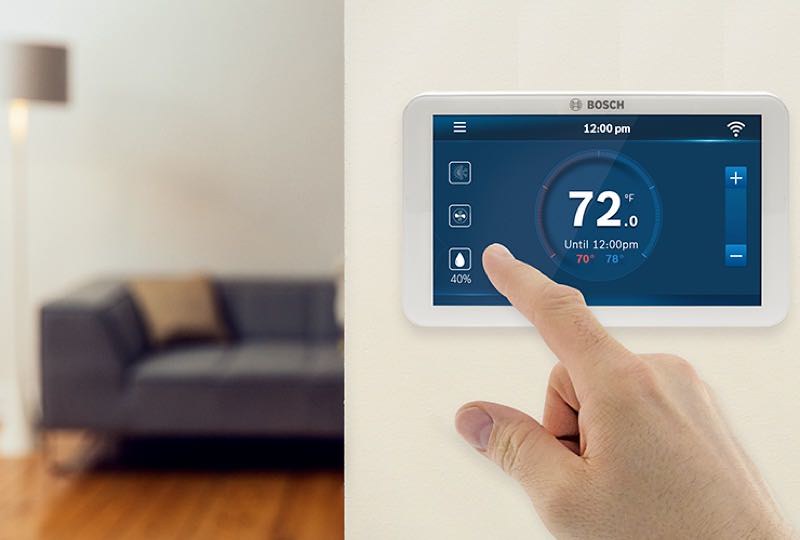On the wall, there is an air conditioning unit mounted, measuring approximately 10 inches wide by 7 inches high, occupying a section about two feet wide. The unit features a prominent digital display with a blue background, which measures around 6 inches wide and 4.5 inches high. 

The top portion of the display has a darker blue background, showcasing several important indicators. At the center, the time is displayed as "12:00 PM" in white, digitized numerals. To the left of the time, there's a wireless signal icon indicating full strength, and to the right, a white hot dog symbol.

Along the left side of the display, three icons indicate the current mode of the air conditioner. At the center, a circular dial shows the current temperature setting as "72°F" in both numeral and text form. Below this, red text indicates "70°F" and blue text shows "78°F," likely representing temperature thresholds or settings.

On the right side of the display, under the wireless signal icon, there are plus (+) and minus (−) buttons. These buttons are connected by a vertical bar, where the plus sign is at the top (north) end and the minus sign at the bottom (south) end, allowing for temperature adjustments.

The entire setup is designed to be both functional and informative, providing a clear and detailed overview of the air conditioning unit's status and controls.